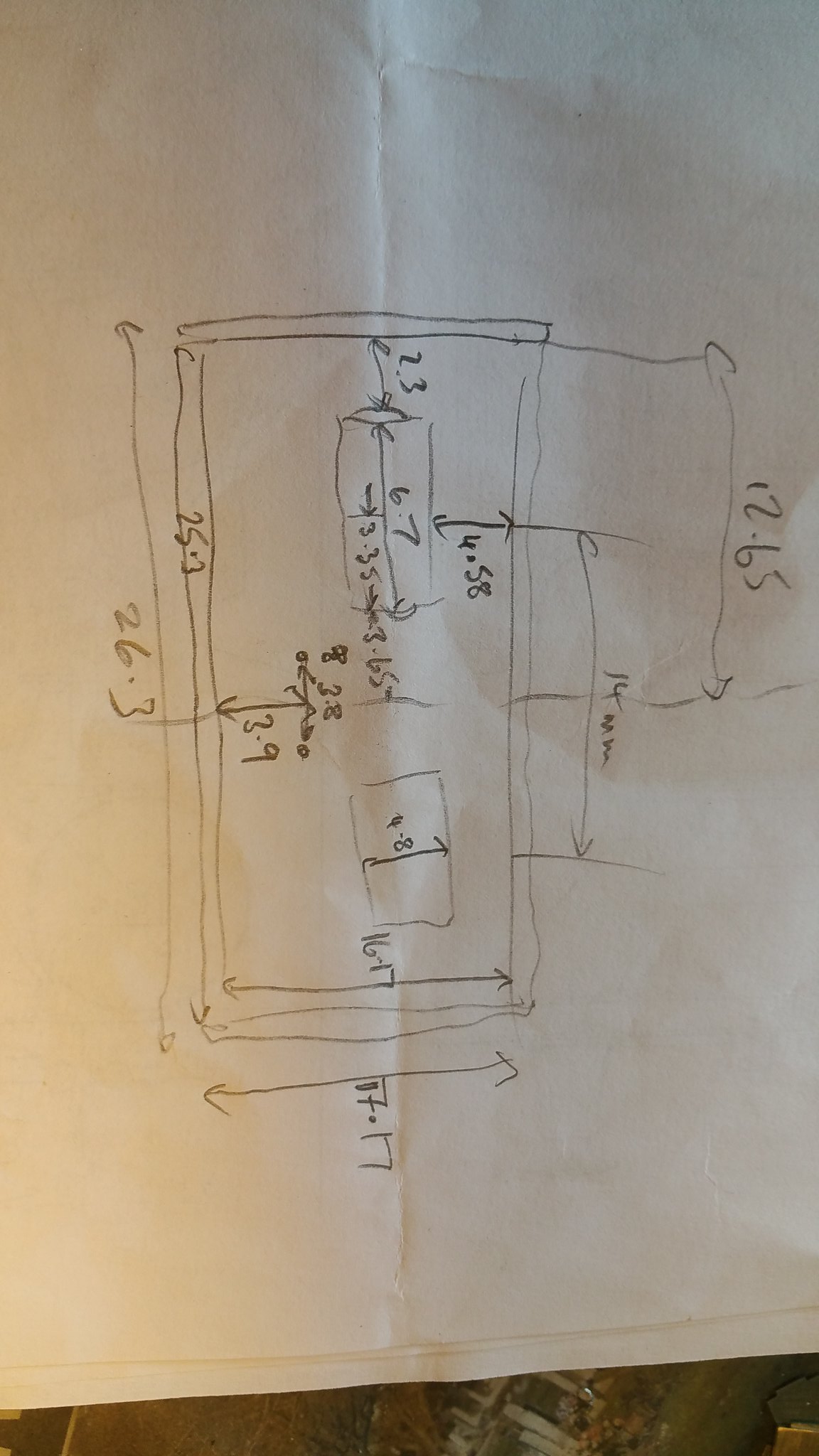The photograph captures a rough pencil sketch on manila paper, depicting the layout of a room within a building. The room, outlined by a double wall, is rectangular with dimensions labeled as 26.3 units in length and 17.17 units in width. Inside the main rectangular space, several smaller rectangles are drawn, each marked with specific measurements. One notable rectangle measures 6.7 units and is positioned 4.58 units away from the right-hand wall. Additionally, there is another rectangle in the lower portion of the drawing, but its measurement is illegible. An extension to the room is visible on the right side, with a long side measuring 12.65 units. There is also a noted but unclear measurement between the centers of two triangles within the main room. The sketch, characterized by its rough and informal appearance, provides a basic floor plan with annotations that are partially difficult to read.